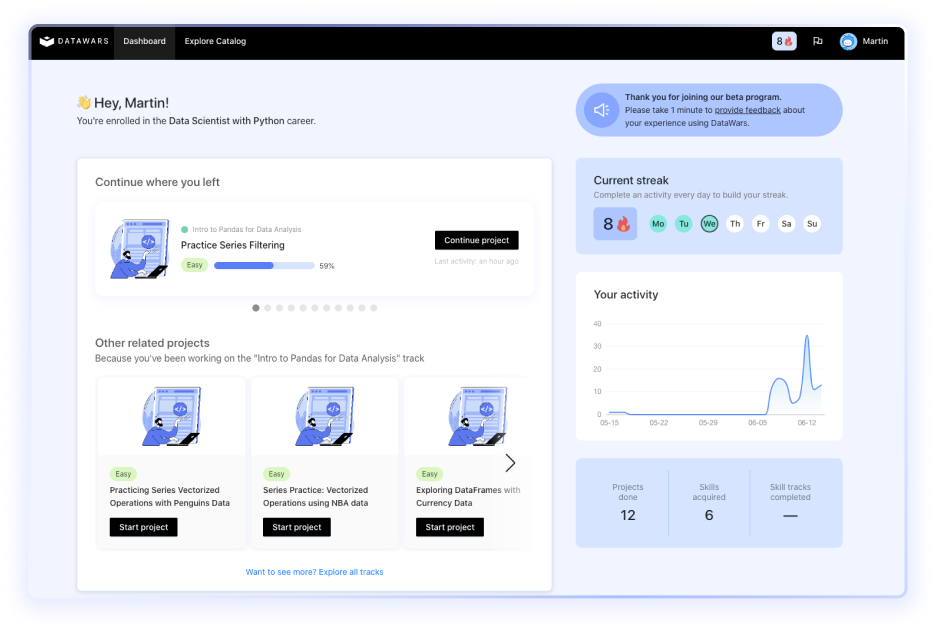This is a landscape-oriented photo of a webpage screen, featuring an aura-like gradient background in light blue shades that intensifies at the top and slightly to the upper left half. Dominating the top part of the image is a black horizontal bar with white text and icons. On the far left, it displays the title "Data Wars" alongside an image or logo. Adjacent to this are navigation options including a highlighted dashboard icon and a link to explore the catalog, both in white.

To the right side of the black bar, a stacked arrangement of icons and elements begins with a light blue box showcasing a fire icon, a flag, and an avatar. The avatar is a light blue circle depicting an alien-like character wearing a headgear labeled "Martin." Below this section, the background transitions to a lighter blue featuring a hand emoji and the greeting, "Hey Martin, you're enrolled in the Data Scientist with Python Career.”

The central portion includes an image of screens, wherein a prominent white box titled "Continue Where You Left" displays a practice series progress bar and multiple options or projects to start. To the right of this, another box titled "Current Streak" features the number eight paired with a fire emoji, accompanied by a chart labeled "Your Activity," likely illustrating Martin's recent engagement on the platform.